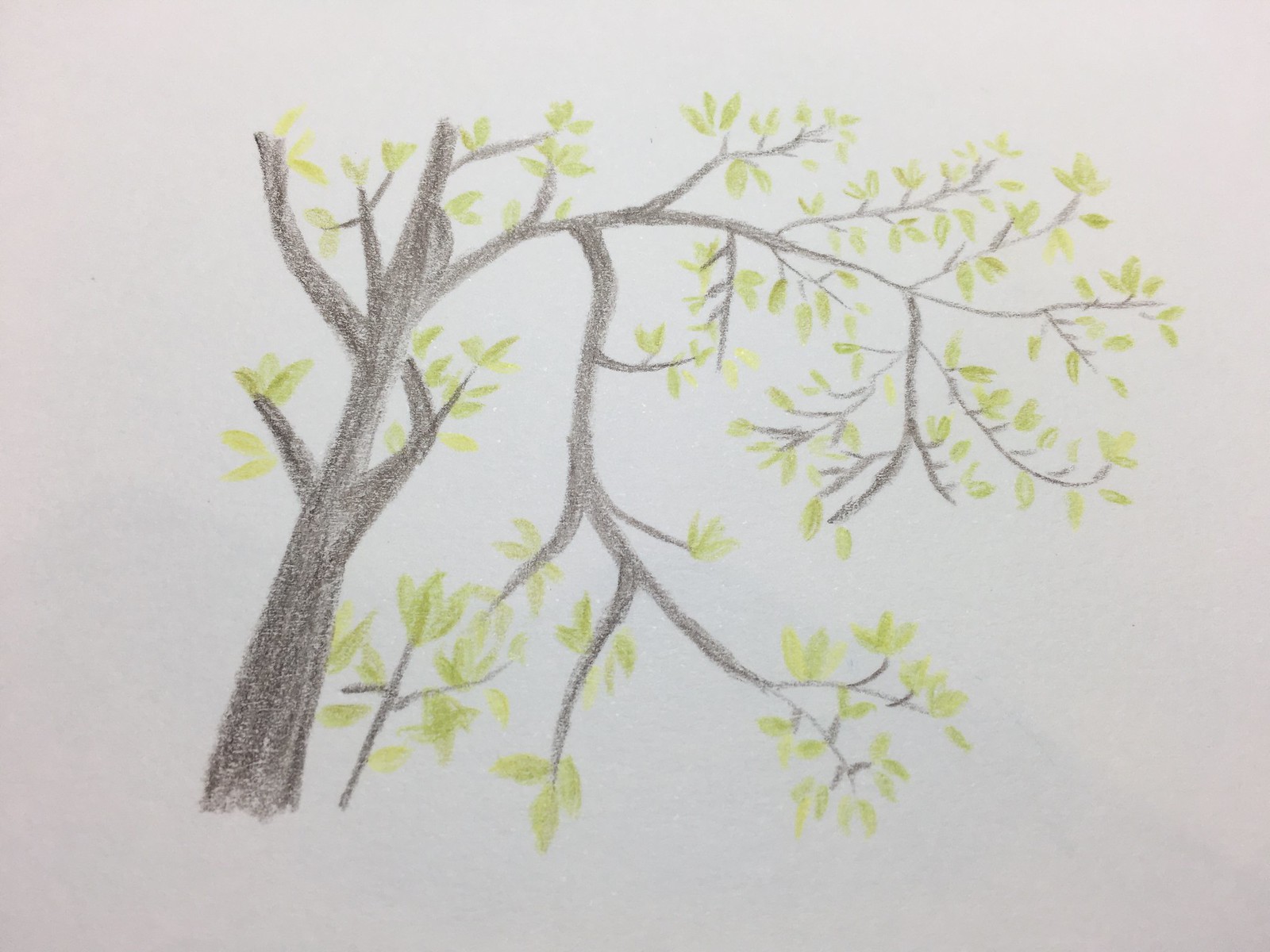A detailed artwork on white paper showcases a tree with intricately shaded black bark, rendered meticulously with a black colored pencil. Branches extend from the trunk, with one curving gracefully to the left and another arching to the right. Numerous other branches, drawn with a green colored pencil, spread out in various directions, adorned with abundant green leaves. Scattered among the leaves are small, white dots that add a touch of texture and contrast to the lush foliage. The overall composition highlights the complexity and beauty of the tree, with its dense network of branches and vibrant greenery.